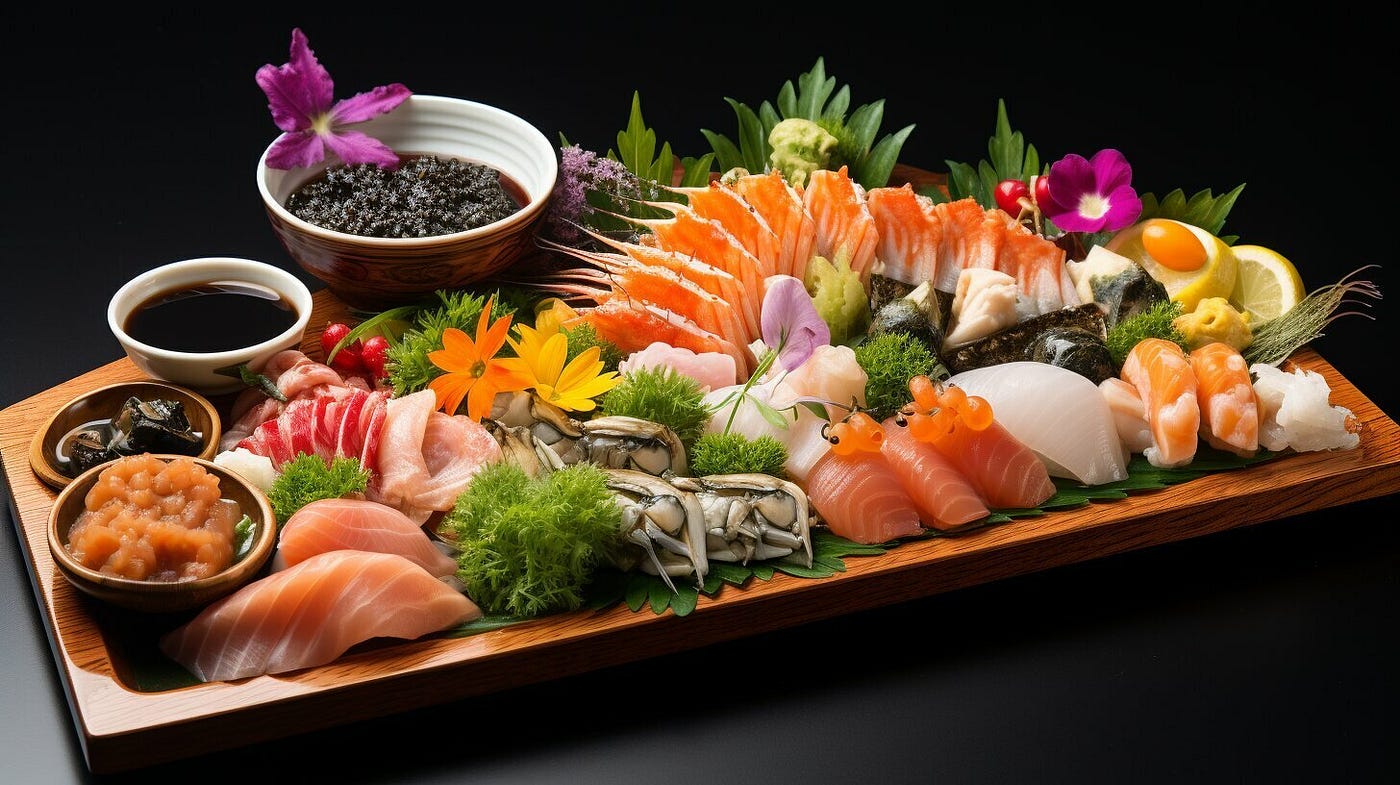A detailed, realistic studio photo showcases an elaborate wooden platter filled with a colorful array of raw seafood, featuring various types of fish, including salmon and shrimp. The wooden tray, treated with a varnish and having a slight indentation in the center, is garnished generously with vibrant greens placed between the seafood. Among the seafood, there are pieces of lemon and an assortment of edible flowers in yellow, orange, and purple, enhancing the presentation. On the left and toward the back of the platter, there are multiple bowls and plates with various dipping sauces, including a dark liquid resembling soy sauce and a mushy carrot-colored dish. Another large bowl, positioned more centrally, contains a dark liquid with what seems to be blueberries. The background is a stark black, and the high-contrast lighting from the left and front highlights the intricate details and rich colors of the arrangement, making it appear very fancy and appetizing.